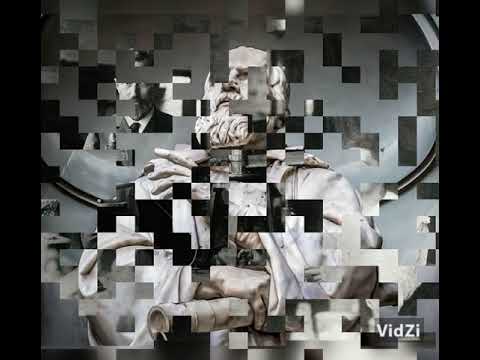The image is a digitally altered artwork featuring a marble statue of an old gentleman in period attire, resembling Victorian-era suits. The statue, which is central to the composition, appears to be looking upwards with one hand reaching out. Overlaying the statue are numerous blocks, squares, and cubes, reminiscent of a QR code or Tetris shapes, that give the image a pixelated and fragmented appearance. These shapes vary in color including white, black, and gray, and sometimes form zigzag patterns and single cubes. To the left of the statue is a partially completed image of a man’s face and shoulders, constructed from these squares, showing only the lower half of his face and a beard. In the bottom right corner, text reads "Vid Z," with both the 'V' and 'Z' capitalized. There are also two black bars running down the sides of the image, framing the overall composition.